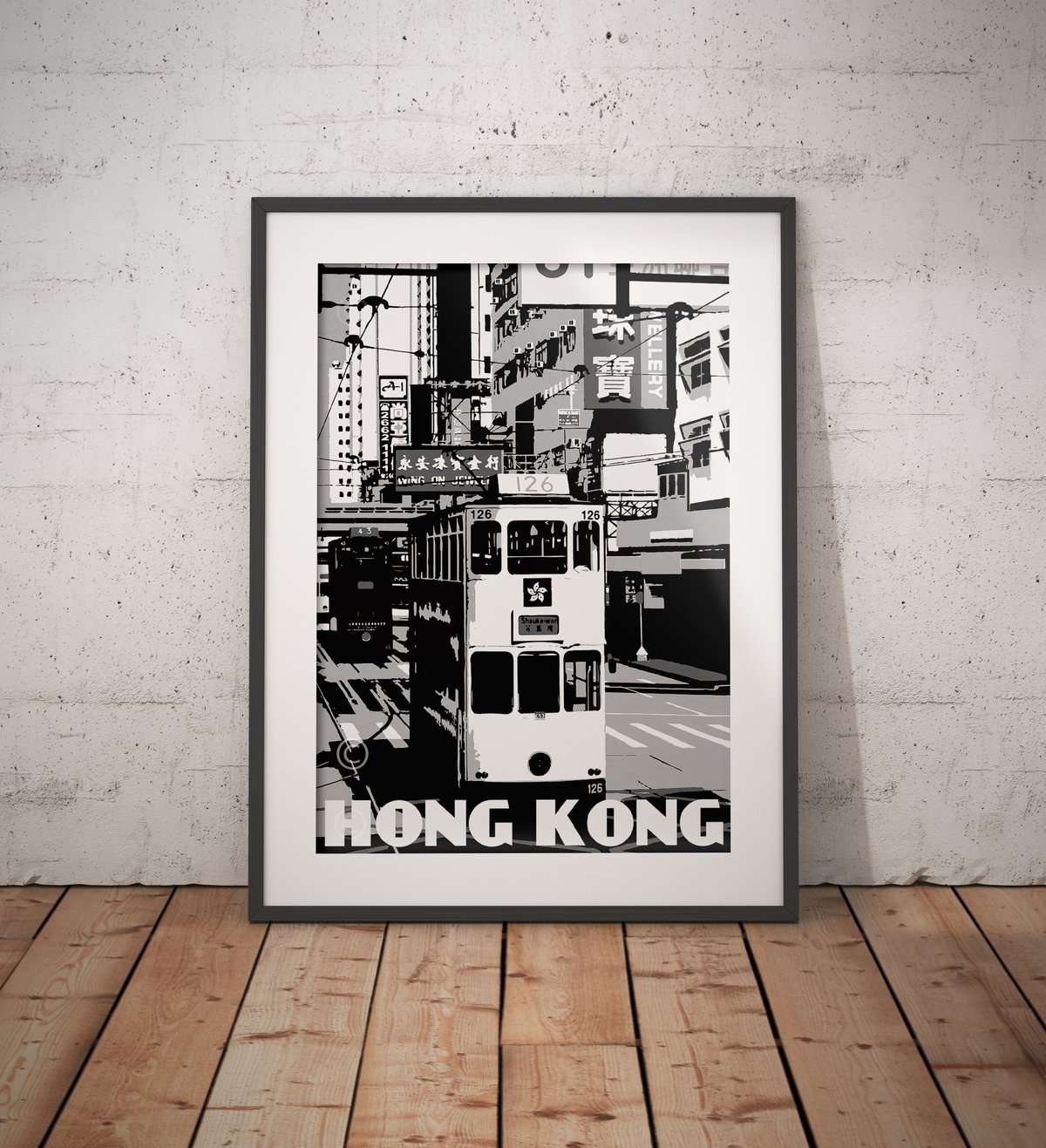In this image, there is a framed piece of artwork leaning against a wall. The frame is a thin, dark gray and features a white matte border surrounding a tall, rectangular black and white print. The print depicts a bustling scene in Hong Kong with prominent vintage tones, featuring a double-decker bus marked with the number 126. The bus is set against a backdrop of city buildings adorned with Chinese signage, and a busy roadway where another double-decker bus can be seen. There's a visible crosswalk and various cars in motion, adding to the urban atmosphere. The text "Hong Kong" is prominently displayed in large white letters at the bottom of the print. The scene captures a lively moment in the city, with intricate details reducing the palette to black, white, and gray tones. The piece is currently resting on a wooden floor, positioned close to a wall, appearing to be ready for hanging.